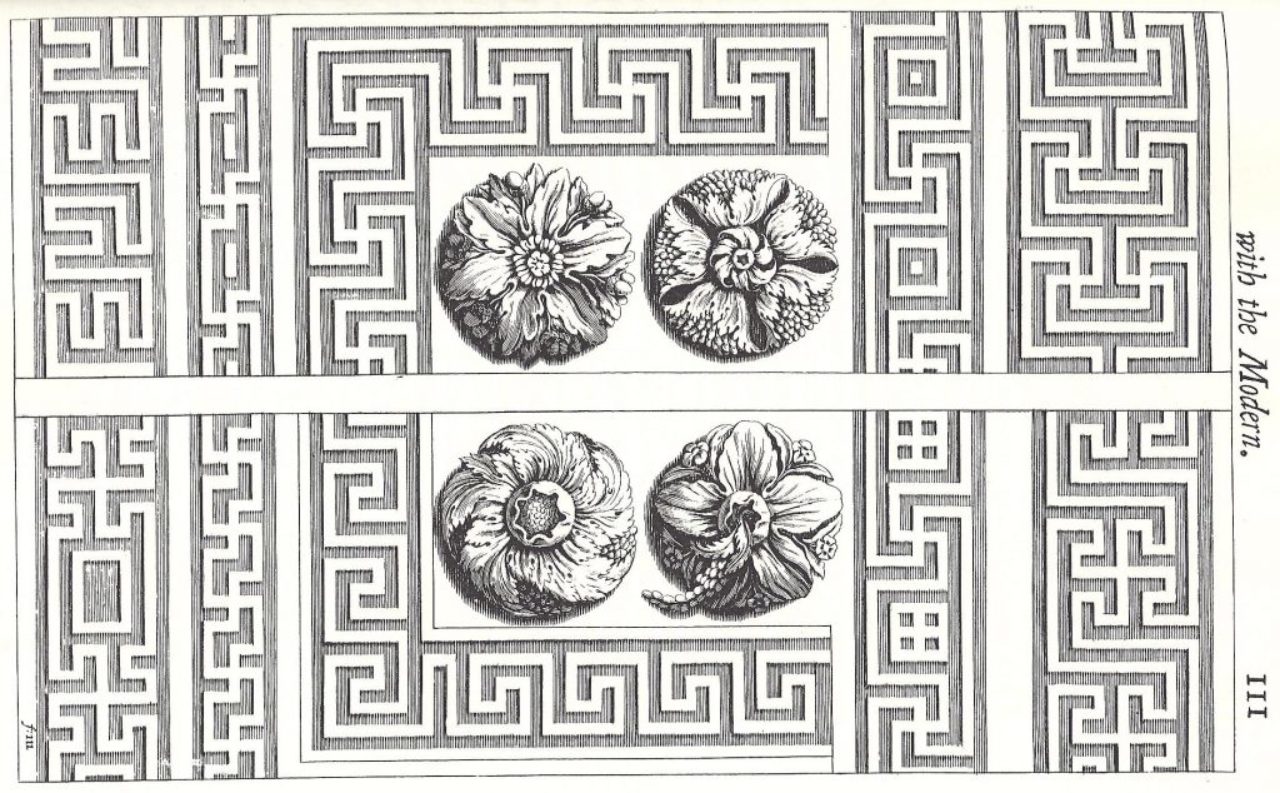The image features a detailed, black-and-white rectangular design dominated by geometric and floral elements. The overall composition is in grayscale, resembling an antique line drawing or engraving. 

The central focus is on four circular, head-on views of flowers, which appear to be sketched. These flowers, though not easily identifiable, include elements that resemble familiar types such as daisies, roses, and sunflowers. Each flower is unique, with distinct characteristics: one has a blueberry-like center, another has feathery petals, the third has hairy petals with nodules, and the fourth has a papery texture. The flowers have been meticulously illustrated to look like stone carvings.

Surrounding this floral quartet is a maze-like, angular pattern created from right-angle turns and geometric blocks. The pattern adds a decorated edging to the image, incorporating various symbols and small intricate details such as dots and squares. 

A horizontal white bar runs through the center of the rectangle, providing a stark contrast to the surrounding design. At the top right corner of the image, there is some text set in italics with serif font, followed by the Roman numeral III (III).

Overall, the image presents a visually striking combination of floral and geometric elements, meticulously crafted to evoke the appearance of traditional engraved wood or printed plates.